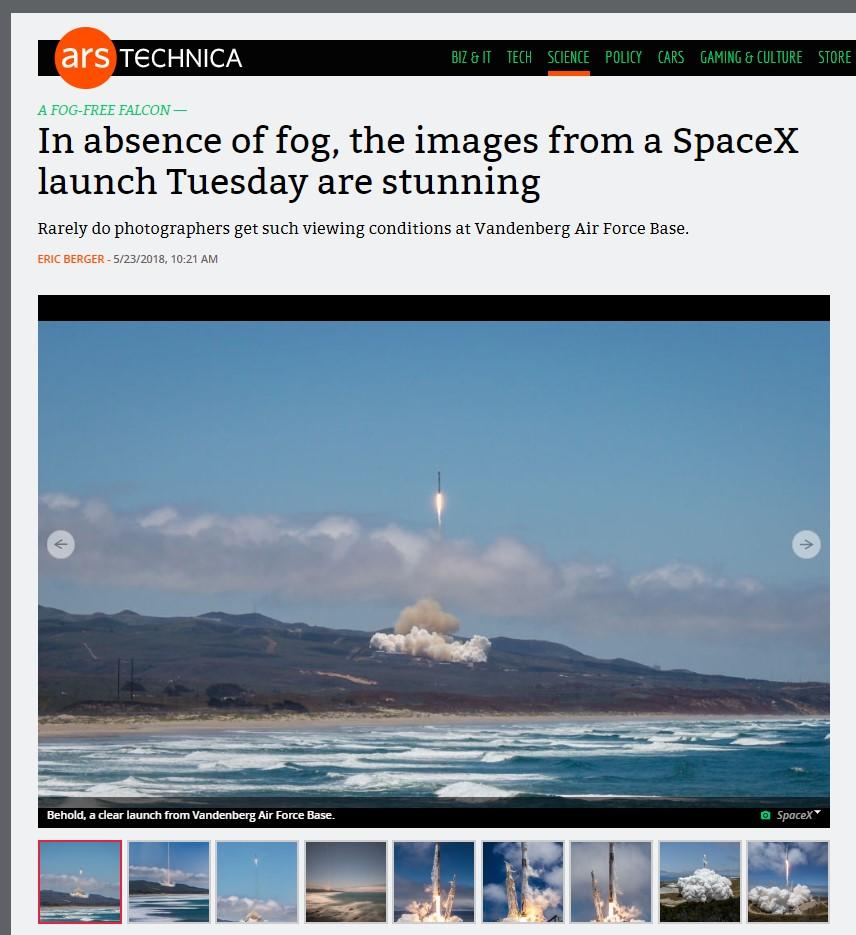This is a detailed caption for an image of an Ars Technica web page, focusing on a science article:

The image depicts a web page from Ars Technica, a renowned technology news and information website. The navigation bar at the top features clickable links highlighted in green, labeled as Biz & IT, Tech, Science, Policy, Cars, Gaming & Culture, and Store. The "Science" tab is currently selected, leading to an article titled "A Fog-Free Falcon." The article describes a SpaceX launch that took place on a clear day, resulting in stunning photographs that are rarely achievable under typical foggy conditions at Vandenberg Air Force Base. The piece is authored by Eric Berger and was published on May 23, 2018, at 10:21 AM. The web page prominently features a main image of a space rocket launch, along with a gallery of nine smaller tiled photos that can be navigated using arrows.